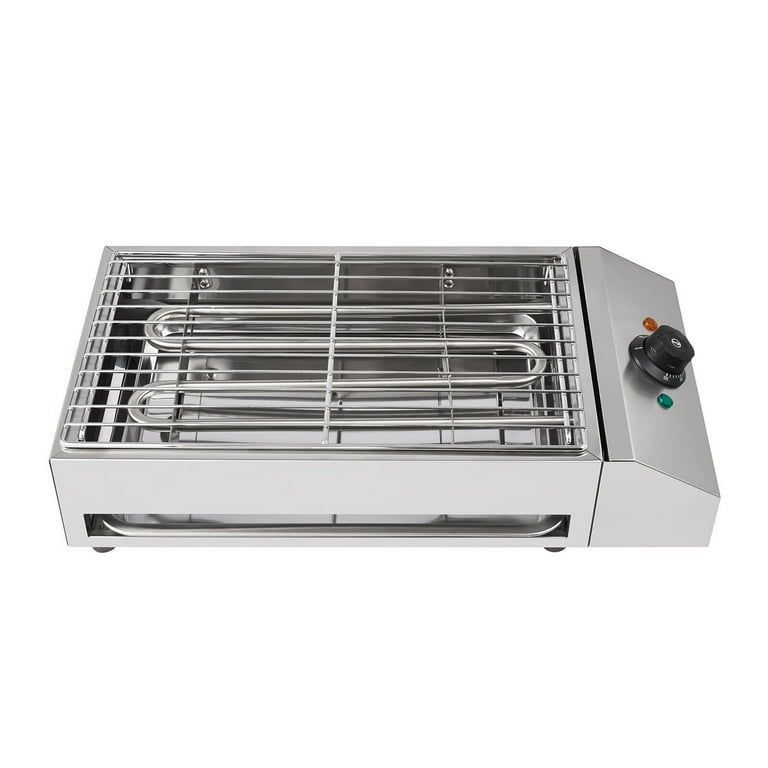The image depicts a close-up of a compact electric grill or heating apparatus, commonly used in a restaurant setting. The device, set against a pristine white background, is constructed from stainless steel and has a rectangular shape measuring approximately 10 inches wide by 5 inches deep. The top surface features an exposed metal grill with a curved coil underneath, serving as the heating element. On the front right side of the grill, there is a control panel equipped with a black dial for temperature settings. Flanking the dial are two indicator lights—a green light on the left and a red light on the right—designed to signal the device's operational status. Additionally, there is a small tray located at the side that can be pulled out and pushed back in. The overall design is clean and functional, aimed at efficient temperature control in a professional kitchen environment.